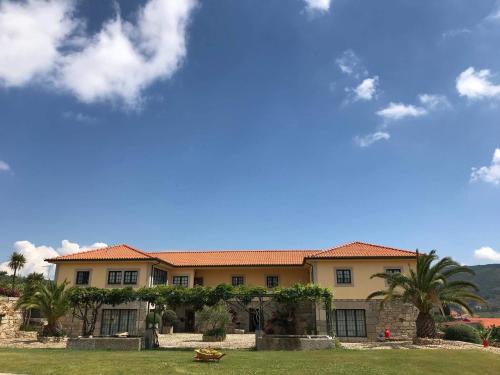The image captures a large, Spanish-style, two-story house with an expansive, green lawn in the foreground. The house features a distinct architectural design with a stone facade on the lower story and light yellow cement walls above. The roof is adorned with red terracotta tiles typical of Spanish tiling patterns. The house is accentuated by multiple windows: nine on the upper level and large glass panel windows on the lower level. Flanking the house are two towering pine trees and several deciduous trees, along with various palm trees around the property, contributing to the lush and verdant scenery. A large sidewalk area runs alongside the house, lined with smaller bushes and cement planter boxes. In the background, rolling green and brown mountains provide a picturesque backdrop under a vivid blue sky dotted with fluffy white clouds.